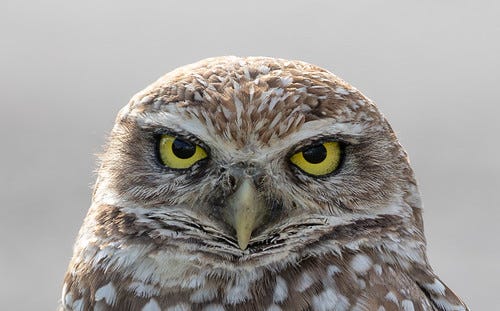This is a sharply detailed photo of a brown owl, captured from about the neck up. Owls generally lack distinct necks, so the focus is strictly on its round, wide head. The owl is facing forward, looking almost directly at the viewer with large, bright yellow eyes that have intense black pupils, giving it a piercing, almost mean expression. A small, bone-colored or yellowish beige beak sits prominently at the front of its face. The feathers are a mix of light brown and white, with small specks of white adding texture to the predominantly brown plumage. The feathers appear particularly detailed, highlighting the owl's intricate feather patterns. There are also white markings above its eyes that resemble eyebrows. The background is a blurry, nondistinct gray, possibly resembling clouds or some other natural setting, which keeps the viewer's attention on the intricately detailed head of the owl. The lighting seems to come from above, casting a slight contrast on the top of the owl's head, making it appear brighter than the rest of its body.